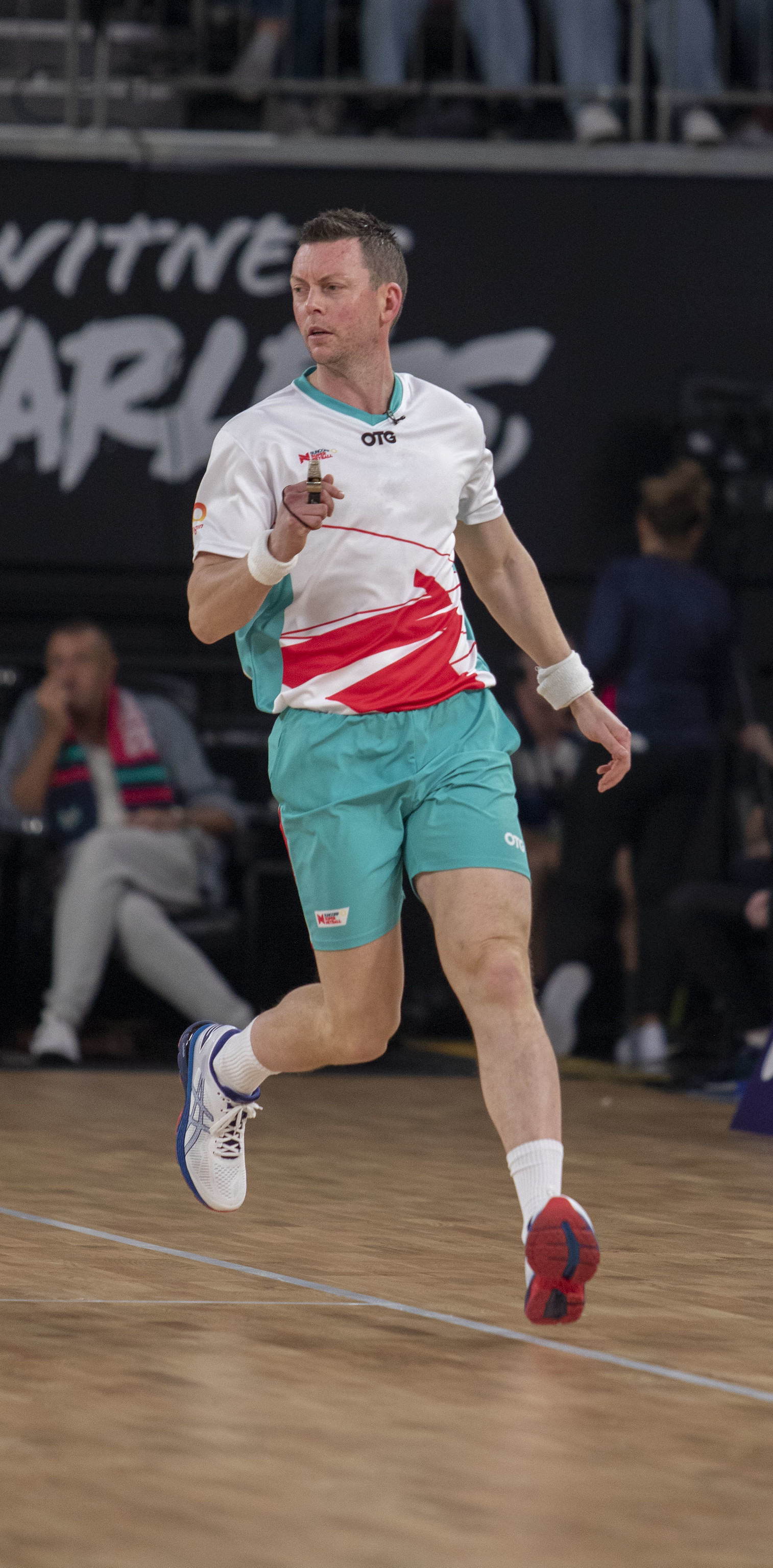The photograph captures a dynamic moment of a white, mid-run sports figure, potentially a referee, in a gymnasium. He is dressed in a white short-sleeved jersey featuring a red swoosh pattern at the bottom and turquoise accents around the collar and sides, paired with light blue shorts and blue sneakers. The gym floor, characterized by its wooden texture and a noticeable grayish stripe, suggests an indoor setting. The individual clutches what might be a whistle in his hand, adding ambiguity to his role. In the background, spectators are visible, some standing, some seated, and the upper sections of the stands reveal only their legs, indicative of a moderately crowded event. A wall with white lettering is partially visible, hinting at the indoor sports venue's vibrant atmosphere. The athlete's focused gaze to the left contrasts with his movement oriented towards the bottom right corner of the frame.